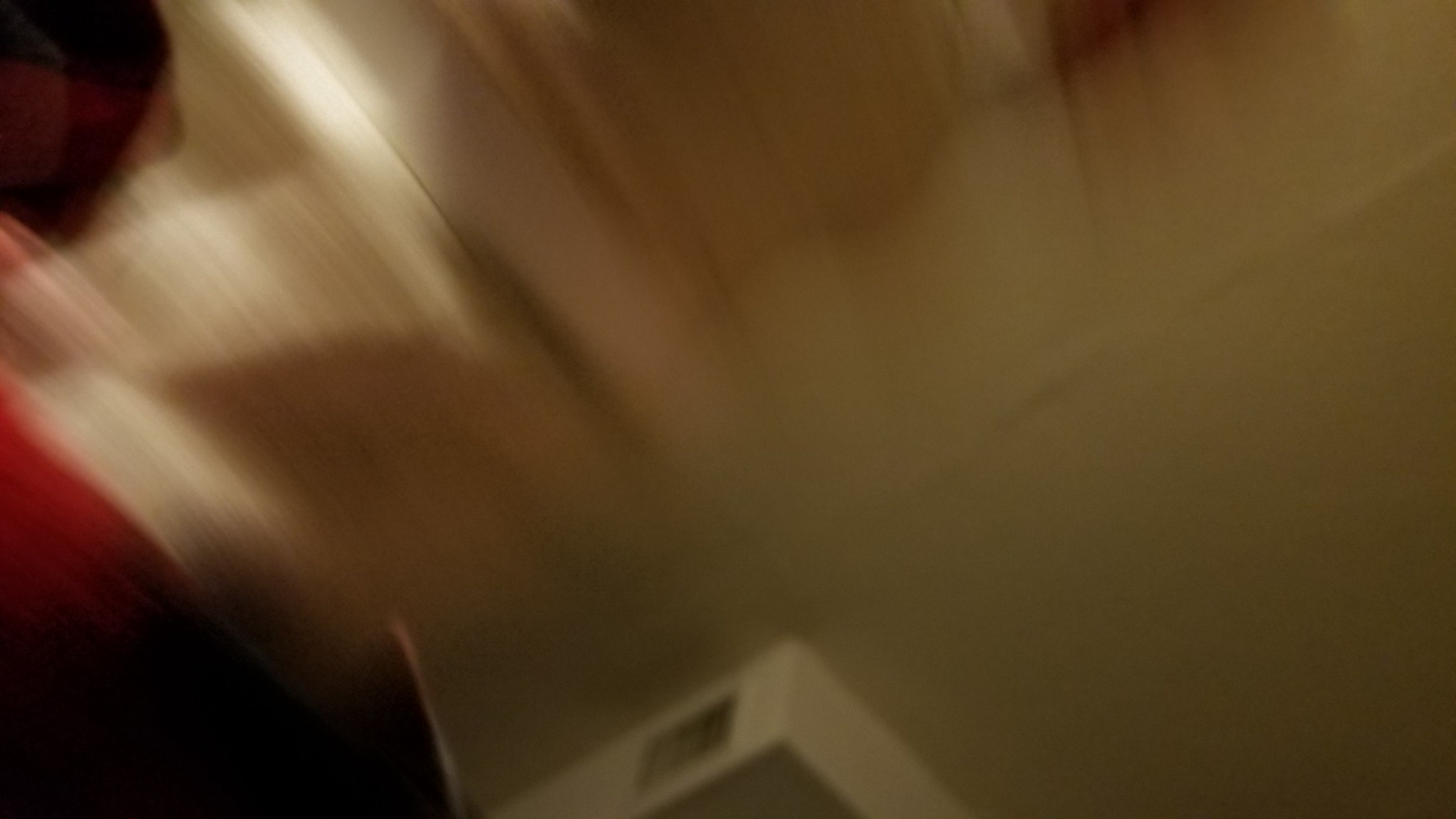This rectangular, landscape-oriented image is entirely blurry, making it difficult to discern specific details. In the upper left corner, there appears to be a window, partially obscured by what seems to be blinds, allowing some light to filter through. Adjacent to this window on the left, a patch of red color is noticeable, which could possibly be due to a curtain or some other decorative element. Dominating the lower-center portion of the image is a white box. The wall behind this box extends upwards towards the right and looks white but is cast in shadow. There also seems to be light pink or light red curtains hanging over the windows, contributing to the appearance of a diagonal line cutting through the image.